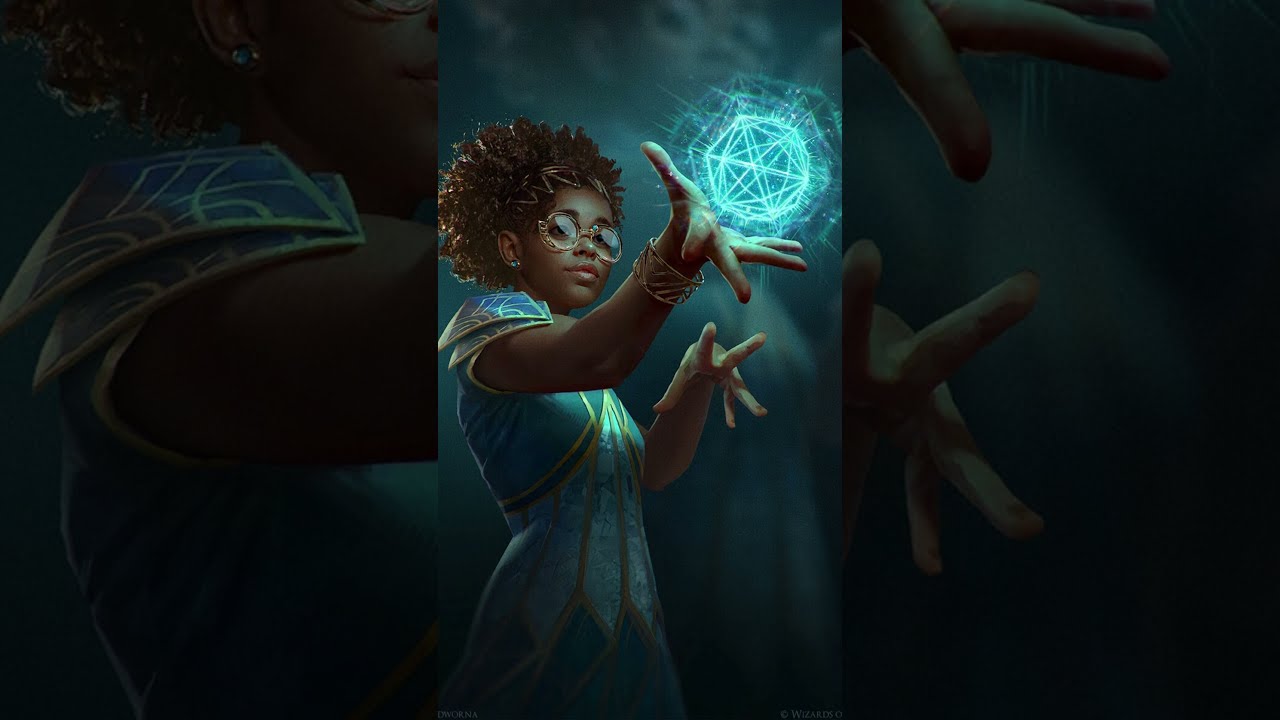In this vivid image, a young black girl is positioned towards the left side, striking a mystical pose reminiscent of Dr. Strange. She wears a blue sleeveless dress adorned with gold and white decorative trim. Her curly brown hair is pulled back, featuring a distinctive zigzag pattern in her bangs, and she sports gold-rimmed glasses reflecting light. The girl's right arm is extended towards the center, with her palm facing up, holding a glowing geometric orb radiating blue light and surrounded by halos, giving it a magical aura. Her left hand points downward, fingers outstretched as if casting a spell. A gold bangle wraps around her right wrist. The backdrop of the image is a cloudy, sci-fi or video game-like setting, with hints of a secondary reflection of the girl visible towards the bottom and left side, enhancing the fantastical atmosphere. The scene seems to be a still shot, likely from a mobile device screenshot, with a palette of colors including brown, yellow, pink, green, blue, and tan.